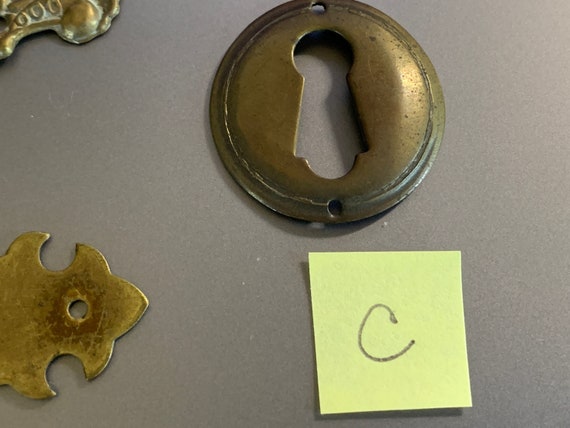This close-up vertical image features a solid gray background and several distinct objects organized with precision. Dominating the top center is a dark gold, almost brown metal disc with meticulously cut details: two symmetrical holes at the top and bottom centers, and a unique internal cutout. The internal cutout begins circular at the top, then angles downwards before extending horizontally and finally curving to a close. Below this disc rests a small yellow square piece of paper, inscribed with the letter 'C' in dark brown or black. Towards the bottom left, there's a dark gold metal leaf design with a circular cutout at its top. This arrangement, resembling a diagram or chart, juxtaposes industrial metallic elements with the simplicity of a handwritten note.